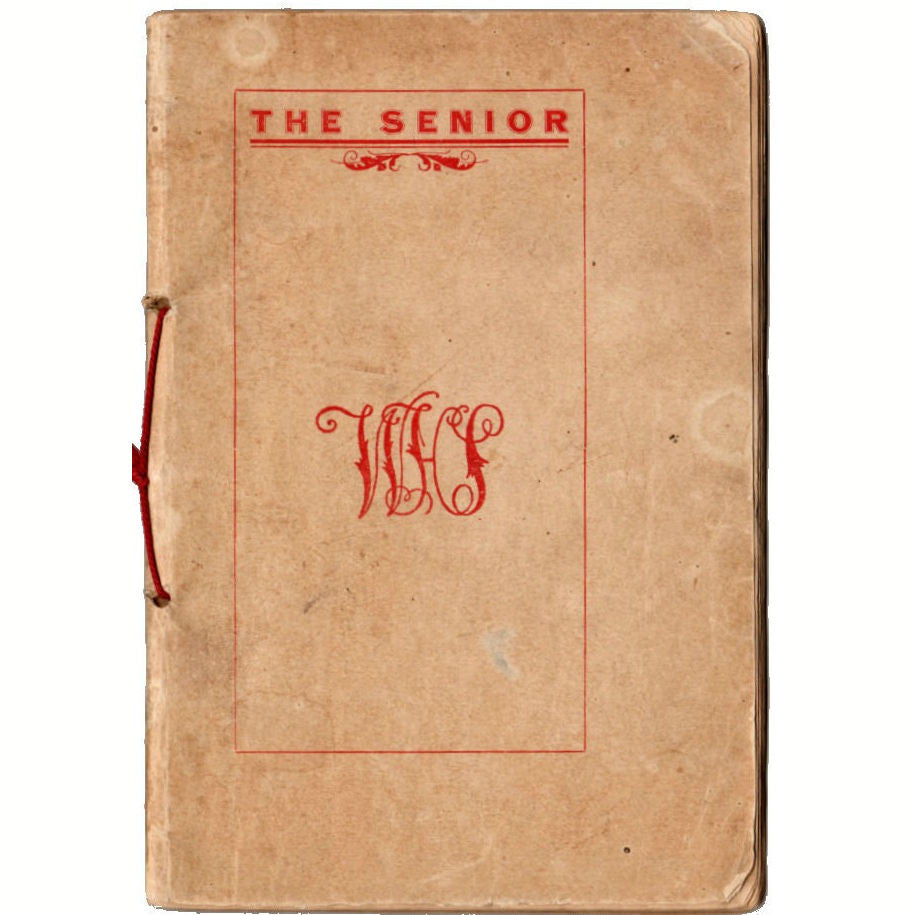This image depicts a highly worn and tattered vintage book with a predominantly brown and tan cover that has aged to a brownish hue over time. The cover features a prominent red rectangle, within which "The Senior" is written in large, red, stylized capital letters at the top. Beneath this, in a highly stylized and cursive script, the letters "WHS" appear, making them somewhat difficult to decipher. The book is bound on the left side with a reddish string or fabric, indicating age and adding to its fragile appearance. The cover corners are notably tattered, with visible stains and splotches suggesting water damage. Despite its deteriorated state, the book exudes a sense of historical significance, possibly serving as a senior yearbook filled with black-and-white photographs, a vintage diary, or a day planner, hinting at its academic or personal nature.